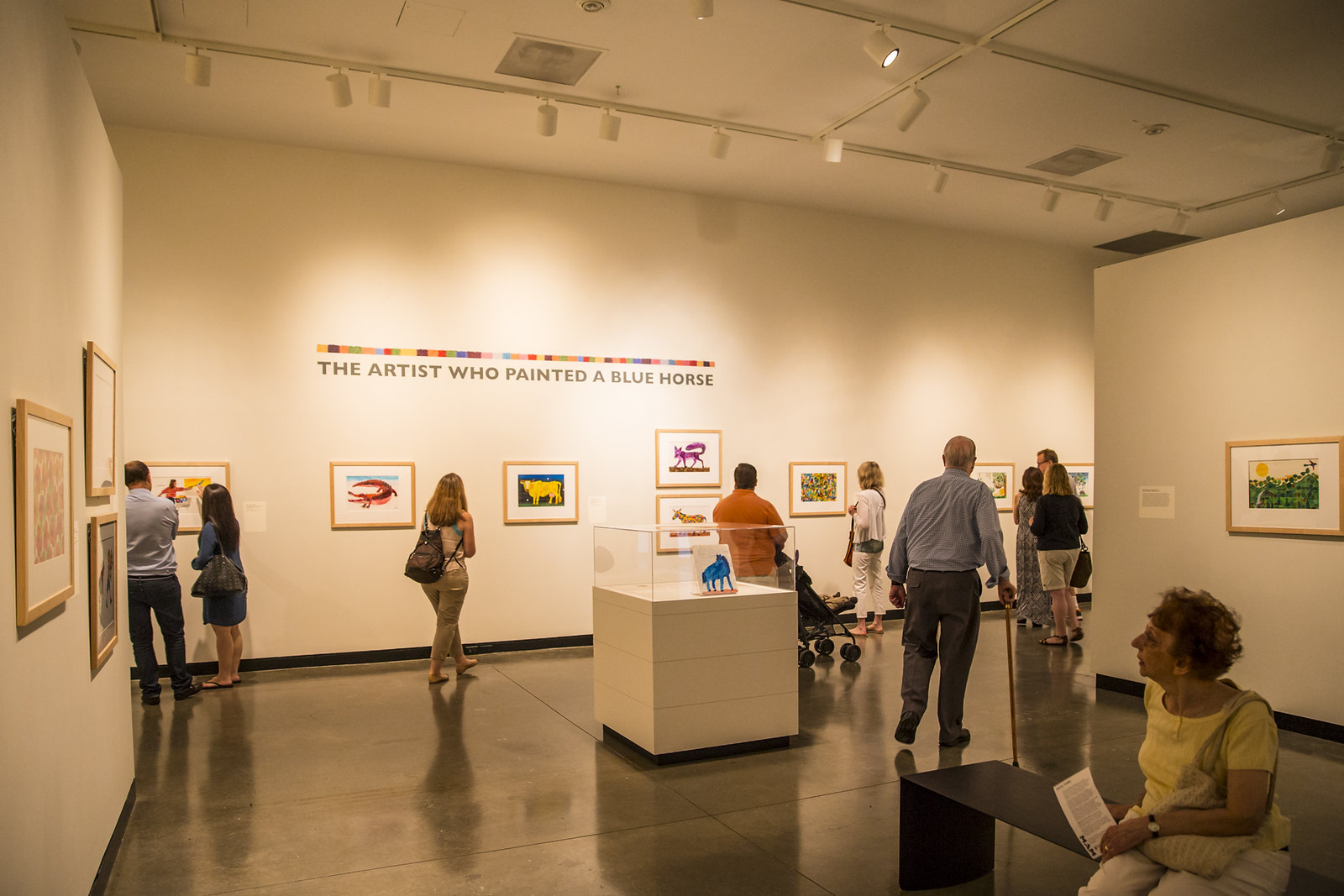The image depicts the interior of a museum exhibit, focused primarily on a corner view towards a back wall. The walls are adorned with a variety of framed, colorful artworks, including a pink and red alligator with its mouth open and its tail curved, a yellow cow or bull, a pink, fuchsia, and purple fox, and a rainbow horse. Below a multicolored thin line and colorful decals, the back wall features the text "the artist who painted a blue horse." The central part of the exhibit features a glass display case containing what appears to be an illustration or painting of the aforementioned blue horse. The museum's lighting is dim, highlighting the white walls and dark khaki-colored floor. 

Several people are seen milling around, observing the artwork. In the foreground, on the right side of the image, a woman with short brown hair, wearing a yellow top, is seated on a dark-colored bench. She holds a program or paper in her right hand and gazes off towards the artworks, with a purse slung over her left shoulder. The overall ambiance is calm, with the focused and varied display of multicolored, imaginative animal paintings and landscapes catching the viewer's eye.